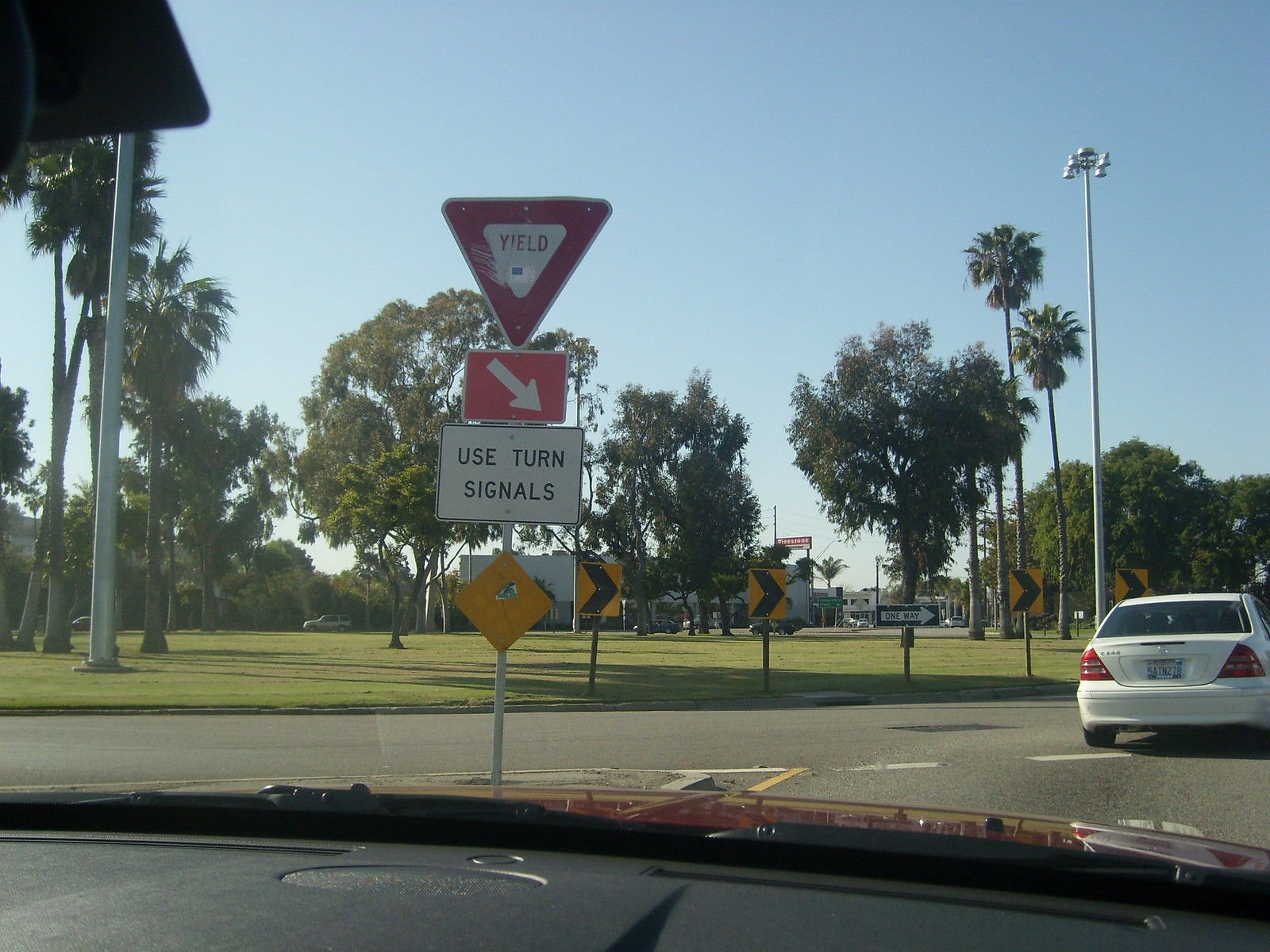A photograph captures a traffic intersection characterized by a traffic circle designed to flow clockwise, indicating it might be located in a country where this traffic pattern is common. Clear signage instructs drivers to yield and use their turn signals. A one-way sign reinforces the direction of travel. 

In the background, a meticulously maintained green field, dotted with palm trees, stretches out, suggesting a tropical or subtropical climate. A towering silver lamppost stands prominently near the roundabout's entry, which appears to be leading into a business district. Although a red sign advertising a business can be seen in the extreme distance, the specific details remain indistinguishable. The foreground features a manhole cover embedded in the pavement, adding a touch of urban detail to the scene.